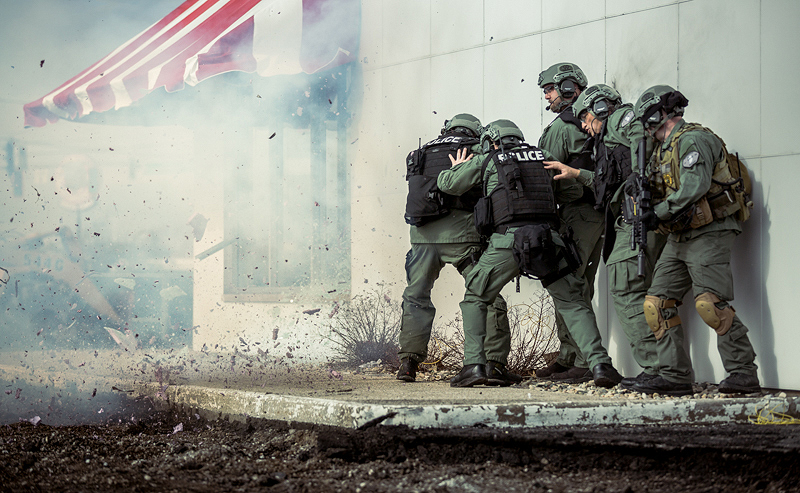This photograph captures a tense moment as five SWAT police officers, dressed in dark green tactical gear with black bulletproof vests labeled "POLICE," stand on a cement sidewalk beside a storefront. The storefront features a striking red and white striped awning, but the most dramatic element is the window beneath it, which has been shattered and blown out, with debris visibly scattering through the air. The officers, positioned to the right of the image, are heavily armed and equipped with knee pads and ear protection. They appear ready and alert, possibly taking cover and preparing for further action amidst what seems like an active explosive event. The composition of the photo starkly contrasts the orderly, lined-up officers with the chaotic aftermath of the explosion, emphasizing the intensity of the situation.